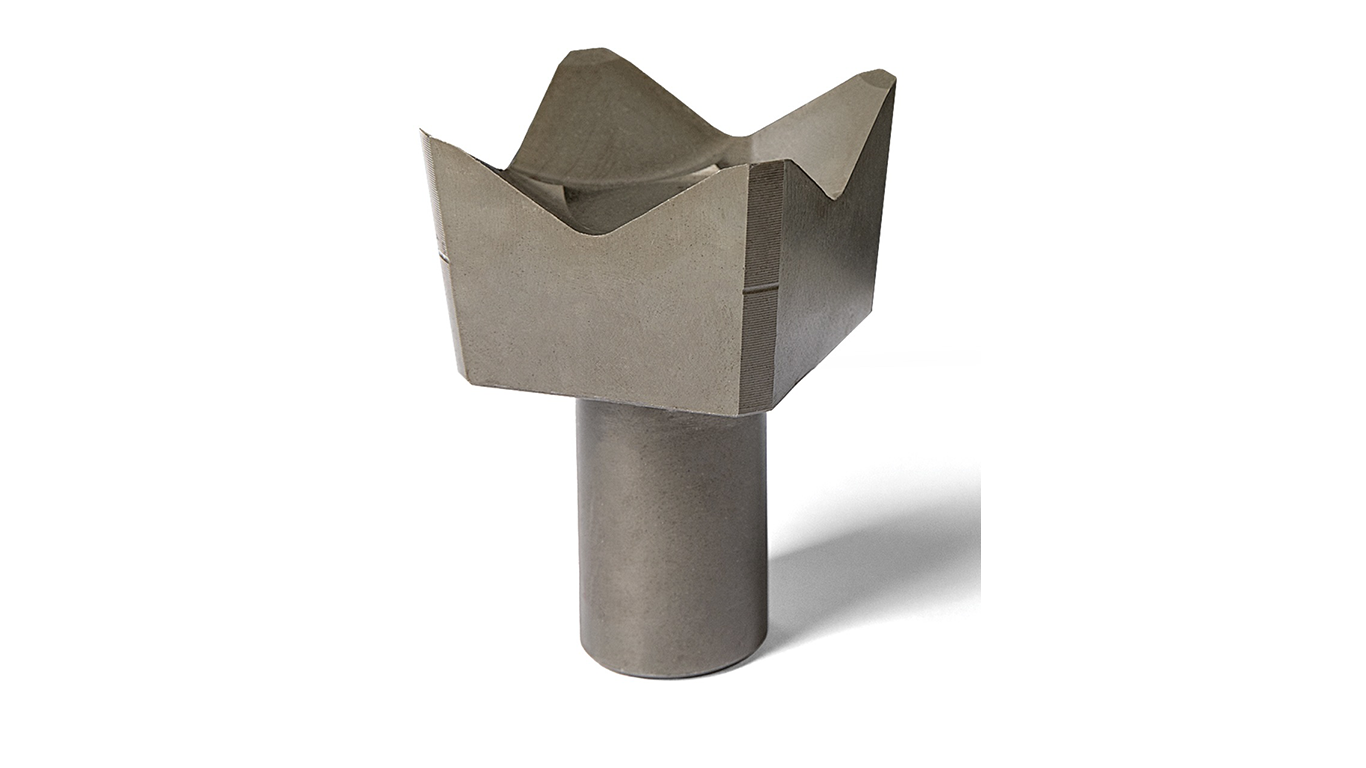The image features a close-up view of a metallic object, resembling a machined component or potentially a piece of abstract hardware. The object is centrally positioned towards the bottom of the frame, set against an empty white background with a slight shadow cast underneath. Its base is cylindrical, extending about halfway up the image, where it transitions into a square-shaped top. The square top has slightly angled corners, giving it a distinctive geometric appearance. The upper surface of the square top curves concavely between each corner, forming arched indentations that descend downward. The object exhibits a gray, metallic finish, suggesting materials like steel or aluminum, and the detailed, flush edges imply it was precisely crafted using machining tools. The overall setting and composition suggest this could be a photograph of a meticulously crafted metallic sculpture or a specialized drill bit head.